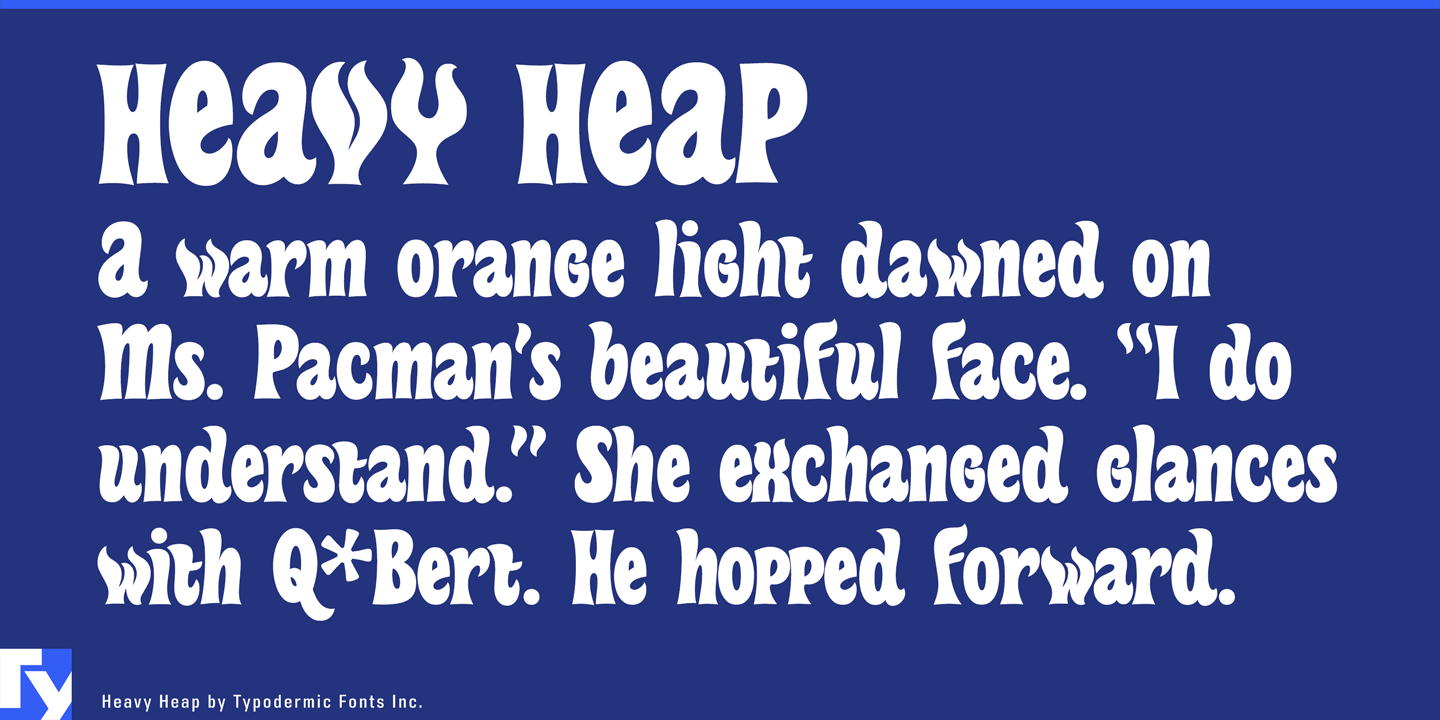The image features a landscape-oriented blue rectangle with a thin lighter blue piping along the top edge. Prominently displayed near the top-left is the title "Heavy Heap" in large, stylized white letters, wherein the 'V' and the 'Y' are designed to resemble flames. Below this, white text reads, "A warm orange light dawned on Miss Pac-Man's beautiful face. 'I do understand,' she exchanged glances with Q-Bert. He hopped forward." In the lower left-hand corner, there's a small light blue square containing the white letters 'TY.' Adjacent to this square, in small white font, is the text, "Heavy Heap by Typodermic Fonts Inc." The overall design is a blend of bold graphic elements and vintage typography.